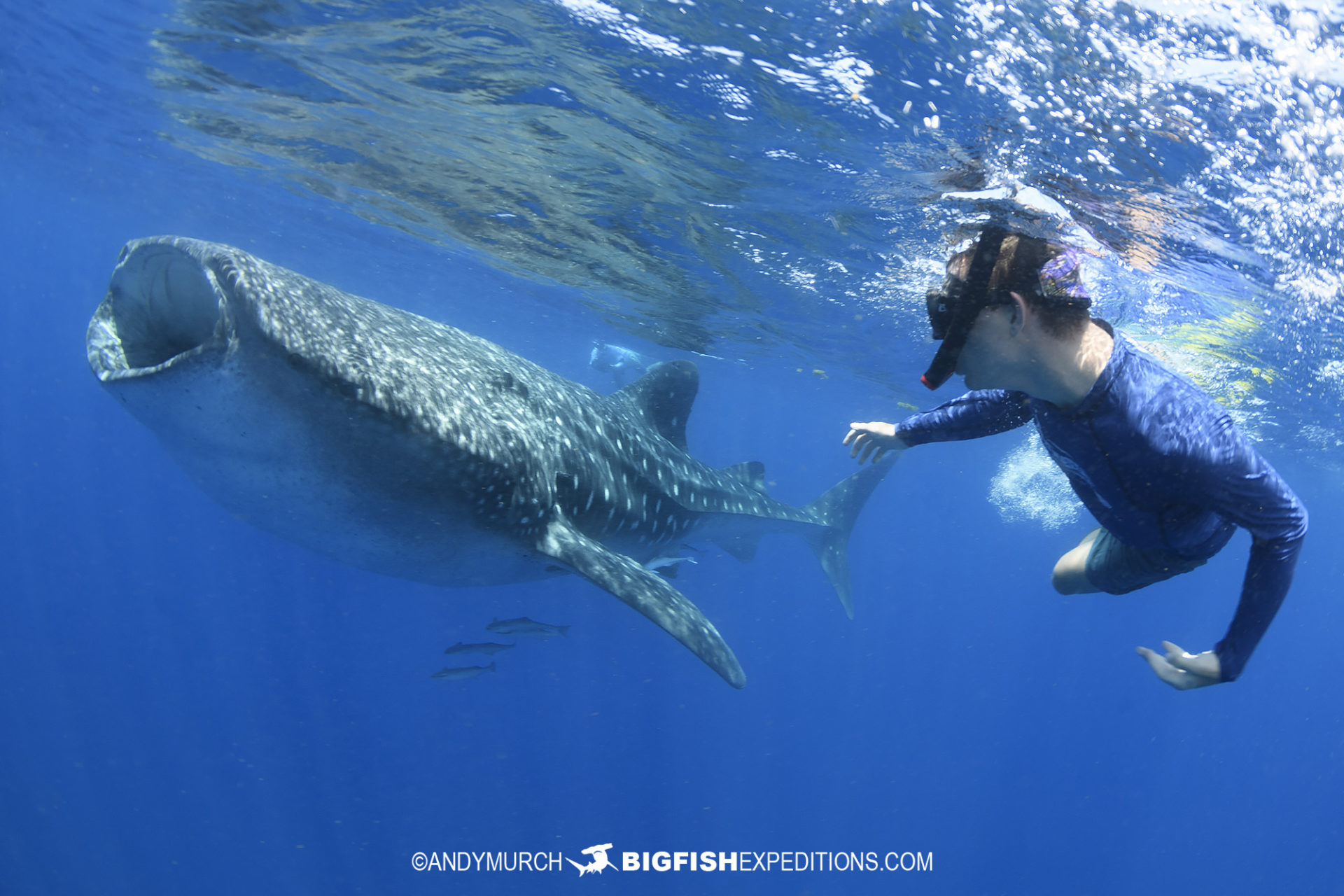This underwater photograph captures a vivid scene with bright blue water, spotlighted by sunlight shining down from the upper right corner where the waterline meets the sky. Dominating the left side of the image is a large whale shark, identifiable by its dark gray speckled upper side and white underbelly. The shark's mouth is wide open, creating a dramatic focal point. Next to it, on the right side of the image, is a diver in a long-sleeved blue shirt and shorts, equipped with goggles and a snorkel. The man is close to the whale shark, reaching out towards it as if to touch it. The diver's head is slightly cresting the waterline. Accompanying this scene, a few small fish can be seen in the background, enhancing the ocean's depth. The bottom of the image carries a watermark that reads "copyright Andy Murch bigfishexpeditions.com".